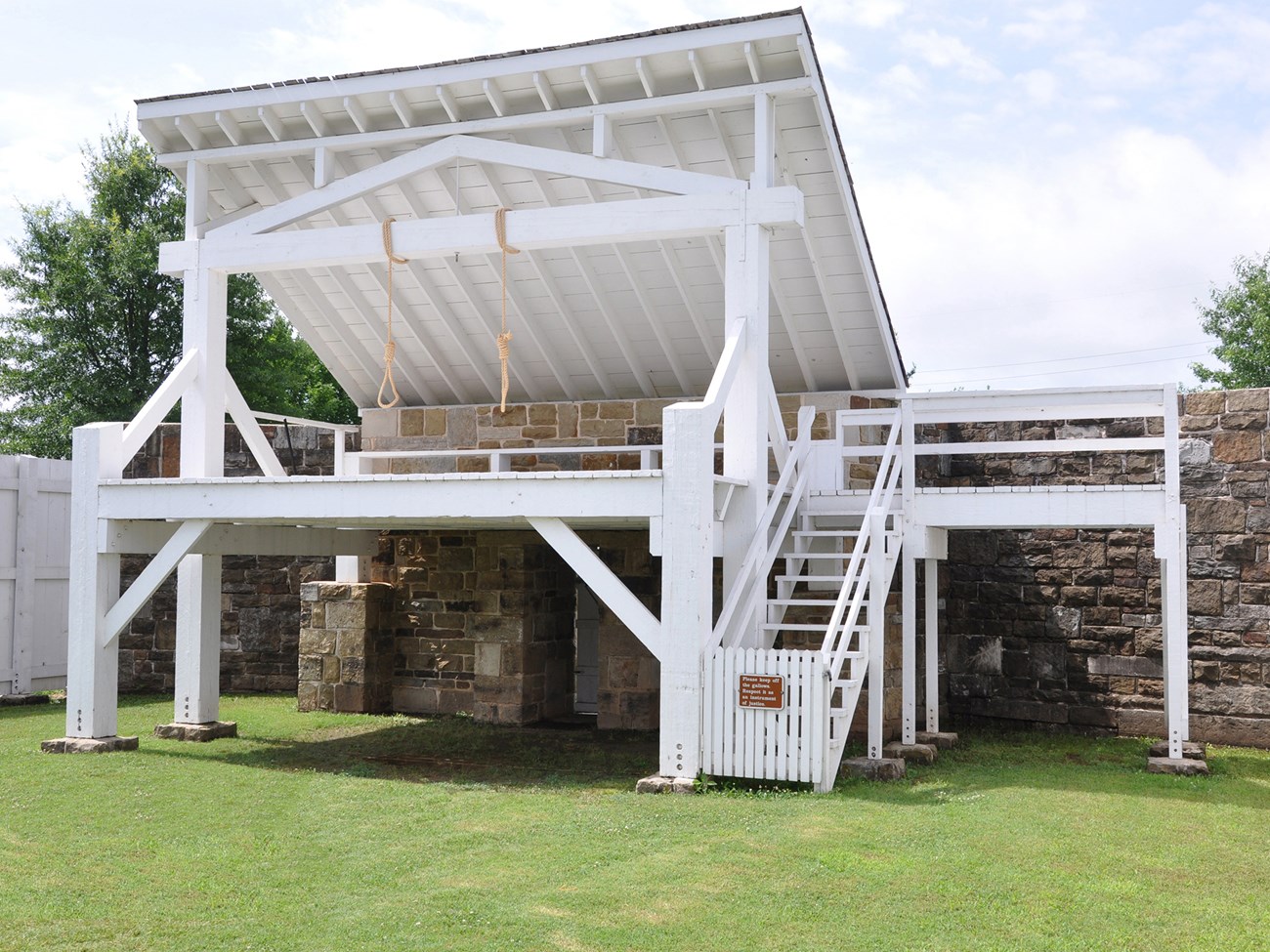The image depicts an outdoor scene under a light blue sky filled with fluffy white clouds. Central to the image is a historical gallows with two hanging ropes, positioned above a white-painted platform accessible by stairs. In the background, there is a tall, red brick wall with lush, vivid green trees peering over its top. Adjacent to this gallows structure is a slanted roof that appears white on the bottom and possibly black on top, supported by a large wooden beam painted white. Surrounding the area is a small white picket fence with a gate bearing a plaque that reads "Please keep off the gallows." The scene is framed by a lush green grassy area, a wall that appears beige, and a further expanse of the white picket fence to the right.